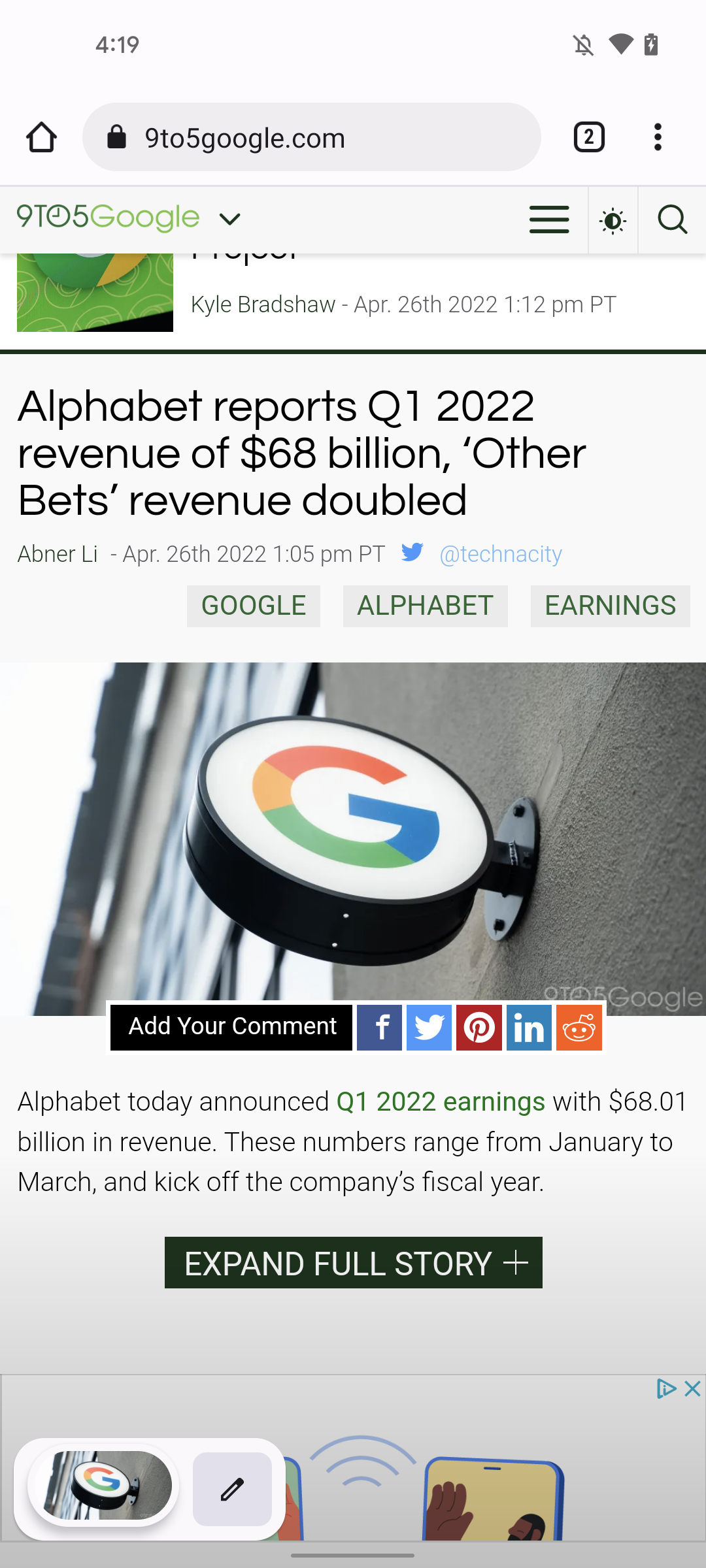This screenshot, captured on a cell phone, features several important details about the device's status and content being viewed. At the top left corner, the time is displayed as 4:19. On the top right, a crossed-out bell icon indicates the phone is on mute. The status bar also shows both the Wi-Fi signal icon and the battery icon. 

In the search bar, the URL "925google.com" is shown, written with the numbers nine and five both spelled out and in numeral form alongside the webpage icon for 925google. The article headline reads, "Alphabet reports Q1 2022 revenue of $68 billion. Other bets revenue doubled." The byline indicates it was written by Abner Lee and published on April 26, 2022, at 1:05 PM PT. 

Beneath the headline, the blue Twitter handle @TECHNACITY is visible, followed by the tag "Google Alphabet earnings." In the main body of the article, a photograph of a circular white sign bearing the Google "G" logo is attached to a building. Below the image, social media icons for commenting and sharing on Facebook, Twitter, Pinterest, LinkedIn, and Reddit are present.

The article reports that Alphabet has announced its Q1 2022 earnings, amounting to $68.01 billion in revenue. This revenue range spans from January to March, marking the start of the company's fiscal year. A call-to-action at the end invites readers to "Expand full story."